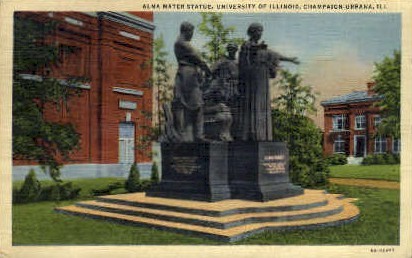This vintage postcard captures the Alma Mater statue at the University of Illinois, Champaign-Urbana. The image features a rust-orange brick building to the left and another similar building to the right, both multi-storied with white windows and doors. The scene is set against a sky with dusty-looking clouds, likely due to the image's age. Surrounding the statue is a lush landscape of green grass, shrubs, and trees, including one notably large tree.

Central to the image is the Alma Mater statue, composed of a woman with outstretched arms, flanked by three other statues behind her, possibly symbolizing students or scholars given their poses. The statues are dark-colored, made of granite or cement, and rest on a platform accessible by three steps. The steps feature gray sides with tan tops. The base of the statue bears an inscription, although the details are not clearly legible in the image.

The overall composition suggests an artist's rendering of a photograph, creating a nostalgic and historic ambiance.